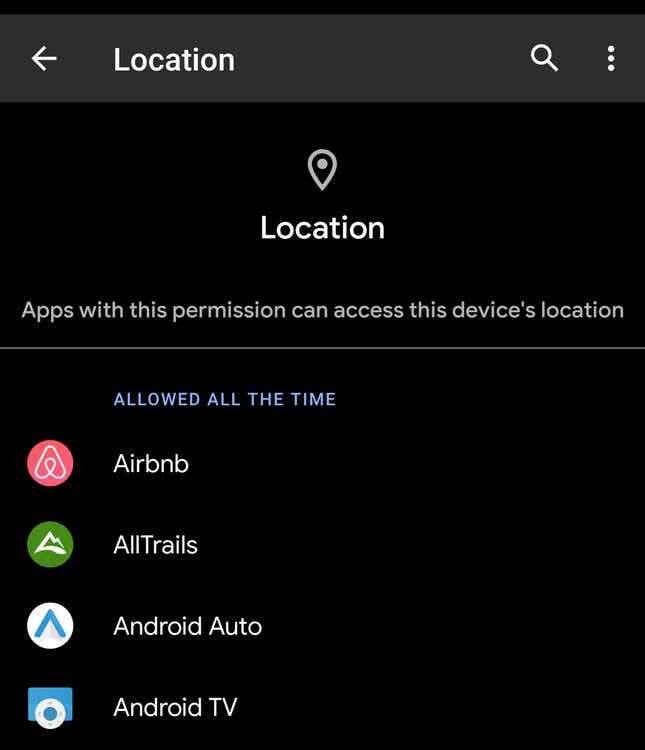The image is a screenshot captured from a smart device, oriented vertically. The background is a solid black, lacking any texture or dimension. At the top of the image, there's a long horizontal gray rectangle overlay. Within this rectangle, there is a left-pointing white arrow, the word "Location" written in white, a magnifying glass icon, and three vertically-aligned dots indicating more options.

Below this bar, the center of the screen displays a location pin icon with the word "Location" in bold white text beneath it. Underneath, a message in gray text reads, "Apps with this permission can access this device's location."

A thin gray line separates this section from a blue label that states "Allowed all the time."

Along the left-hand side of the image, a list of app icons that have location permissions is visible:
1. A red circle with the label "Airbnb."
2. A green circle with the label "AllTrails."
3. A white circle with an upside-down V-shaped icon labeled "Android Auto."
4. A blue rectangle with a white circle on top labeled "Android TV."

This image appears to be a screenshot of a device's location permissions settings screen.